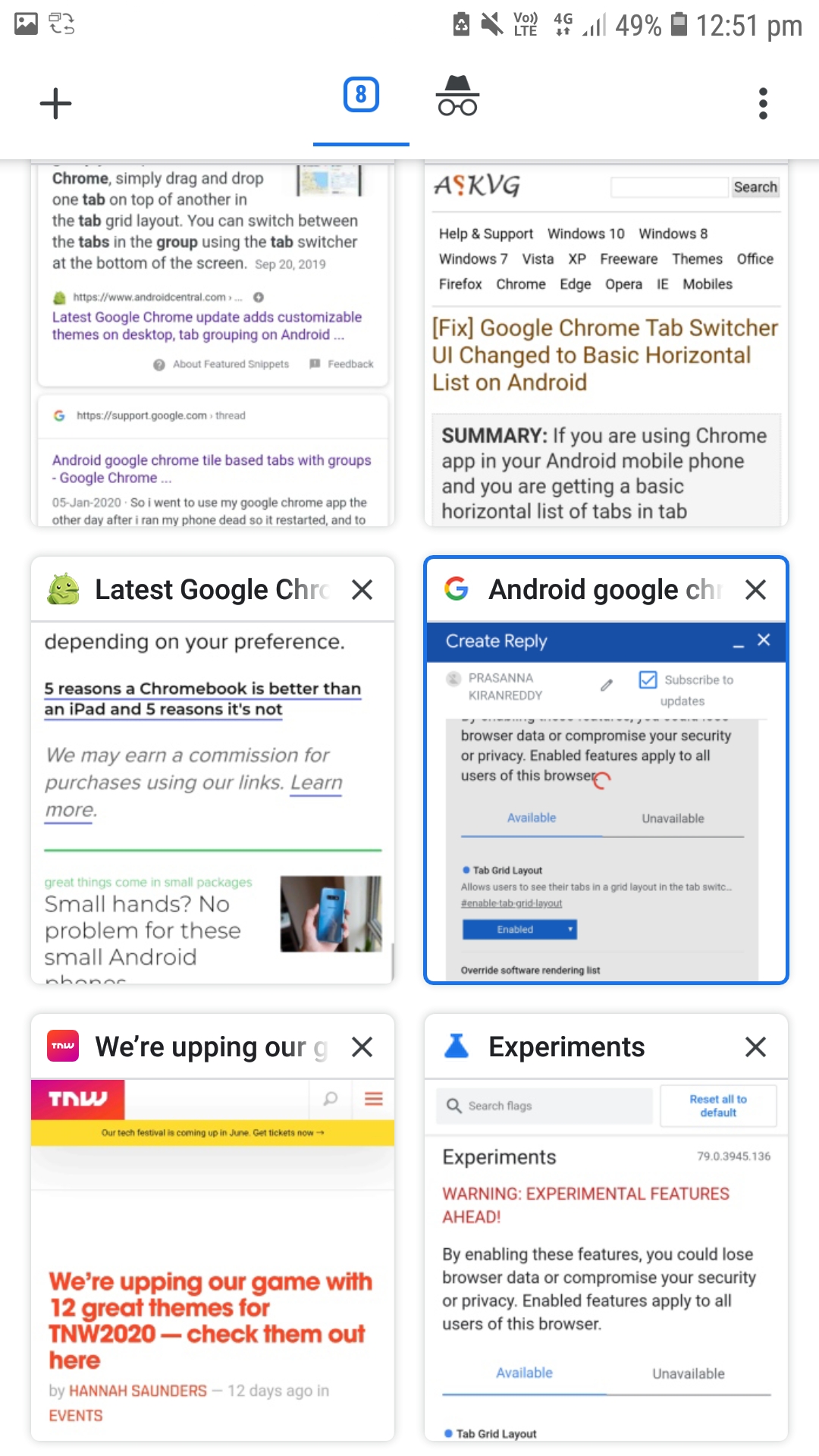A detailed image caption for the provided voice description:

"This is a screenshot of a smartphone’s screen showing the status bar and a webpage in tile view on the Chrome browser. In the status bar, there are icons indicating a photo gallery, a muted volume, a partial 4G network signal, a 49% battery level, and the time which reads 12:51 PM. 

The visible webpage tiles contain various articles and features related to Google Chrome and Android. The first tile discusses the latest Google Chrome update, which includes customizable themes for the desktop and tab grouping on Android. The second tile addresses a UI change for Google Chrome tabs, switching to a basic horizontal list on Android. The third tile compares the advantages and disadvantages of Chromebooks versus iPads, listing five reasons for each. 

The fourth tile, which is currently selected, is a reply form titled 'Android Google' apparently for some service. The fifth tile promotes an event, TNW 2020, highlighting 12 new themes. The sixth and final tile gives a warning about experimental features, cautioning users about potential instability. All these tiles pertain to the Google Chrome browser."